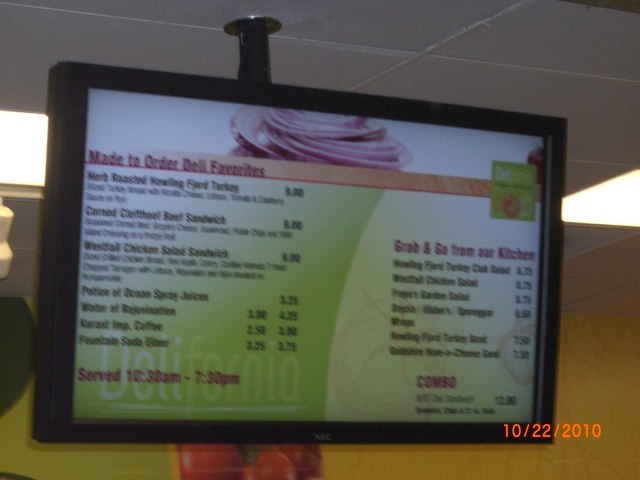This photograph captures a widescreen monitor suspended from a white-grey rectangular sectioned ceiling by a black post. The screen, encased in a black bezel, prominently displays a menu. Behind the screen, a yellow wall can be discerned. The menu shown on the screen features several textual elements: at the top, there’s a blurred, partially visible pink soft-serve ice cream graphic. Below, in bold red text, it reads, "Made to Order Deli Favourites." The middle section contains a list of menu items in black text with detailed descriptions and corresponding prices, though the details are blurred and indistinct. Following this, another red text block states, "Served 10:30am to 7:30pm." On the right side, red text announces, "Grab and Go from Our Kitchen," followed by another list of items and prices in black text. In the bottom right corner, a red heading reads, "Combo," with a single item and its price listed beneath.